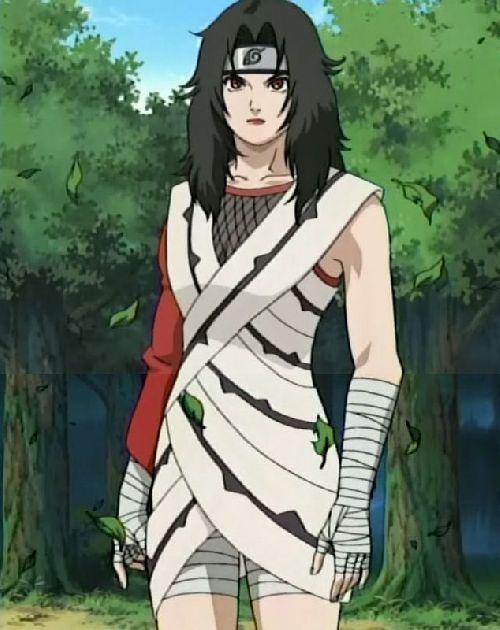The image depicts a female cartoon character standing in a lush, forested environment. The character has black, long hair and is adorned with a silver headband featuring an insignia. She has brown eyes, a small mouth, and her expression is directed straight ahead. She's dressed in a white outfit with brown lines, resembling a dress, and also has bandages wrapped around her forearms, hands, and legs, giving her a warrior-like appearance. Her exposed hand up to where the bandages begin contrasts with her other fully covered, red-sleeved arm. Green leaves are falling around her and resting on her outfit, while two large trees with abundant green foliage dominate the background, against a backdrop of a blue sky.